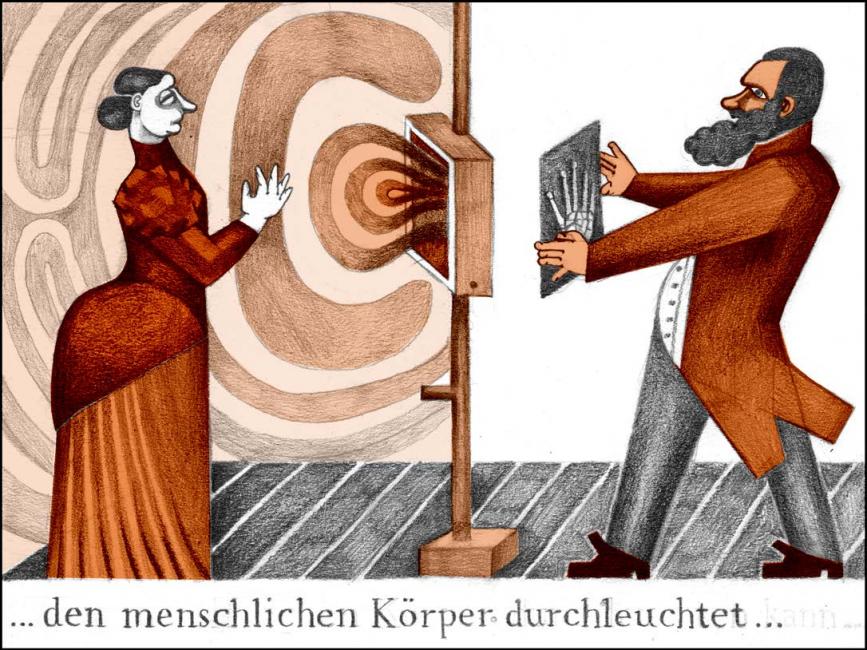A vintage, stylized illustration depicts an early radiography procedure, reflective of late 19th to early 20th-century fashion and technology. On the left, a pale-skinned woman with a long, pointy nose and big eyes is dressed in a high-necked, red Victorian dress with her black hair styled in a bun. She stands with her right hand against an old x-ray machine, characterized by a central brown box emanating expanding concentric circles, possibly representing radiation. Shadows from the machine extend towards her. Opposite her, on the right side, stands a man with a dark beard and short cropped hair, dressed in a brown blazer similar in color to the woman's dress, white button-down shirt, gray pants, and brown shoes. He holds up an x-ray film of a hand towards the light source from the machine, examining it intently. The background to the right is white, while the left side shows varying shades of brown. German wording, interpreted as "den menschenschen körper durchlustet," appears at the bottom of the illustration. The overall color scheme is muted, enhancing the vintage and scientific ambiance of the scene.